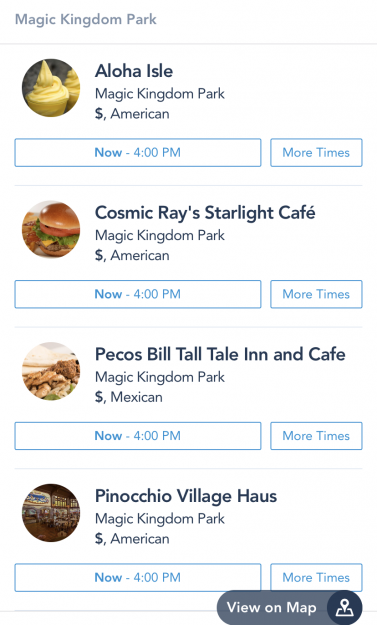The image displays a detailed list of dining options at Magic Kingdom Park, organized in a structured format with various graphical elements. At the top, a gray header reads **"Magic Kingdom Park"**, followed by a gray line. Below that, there are several sections, each denoting different eateries with accompanying icons and text.

1. **Aloha Isle**: 
   - Beside a cupcake or ice cream icon
   - Text in black font reads: **"Aloha Isle, Magic Kingdom Park, $" (American)**.
   - A blue square with white background beneath it states: **"Now – 4 PM"**.
   - A neighboring blue square indicates: **"More times"**.

2. **Cosmic Ray’s Starlight Café**: 
   - Accompanied by a hamburger icon with a brown bun.
   - Black font text reads: **"Cosmic Ray’s Starlight Café, Magic Kingdom Park, $" (American)**.
   - Below, a blue square on a white background reads: **"Now – 4 PM"**.
   - A similar adjacent blue square mentions: **"More times"**.

3. **Pecos Bill Tall Tale Inn and Café**: 
   - Represented by a fries icon.
   - Text in black font states: **"Pecos Bill Tall Tale Inn and Café, Magic Kingdom Park, $" (Mexican)**.
   - Blue square beneath reads: **"Now – 4 PM"**.
   - Another blue square next reads: **"More times"**.

4. **Pinocchio Village Haus**: 
   - Indicated by a distant, indiscernible icon.
   - Black font information says: **"Pinocchio Village Haus, Magic Kingdom Park, $" (American)**.
   - Blue square with white background below it reads: **"Now – 4 PM"**.
   - Adjacent blue square indicates: **"More times"**.

Additional elements:
- A gray line runs underneath the last entry.
- Mixed into this gray line, on the right side, is a gray circle with white text saying: **"View on map"**.
- Nearby is a black circle featuring a white circle and a white square beneath it, though its details are unclear.

This caption transforms the voice-described information into a detailed, structured description, clearly presenting the details of the image for greater clarity.